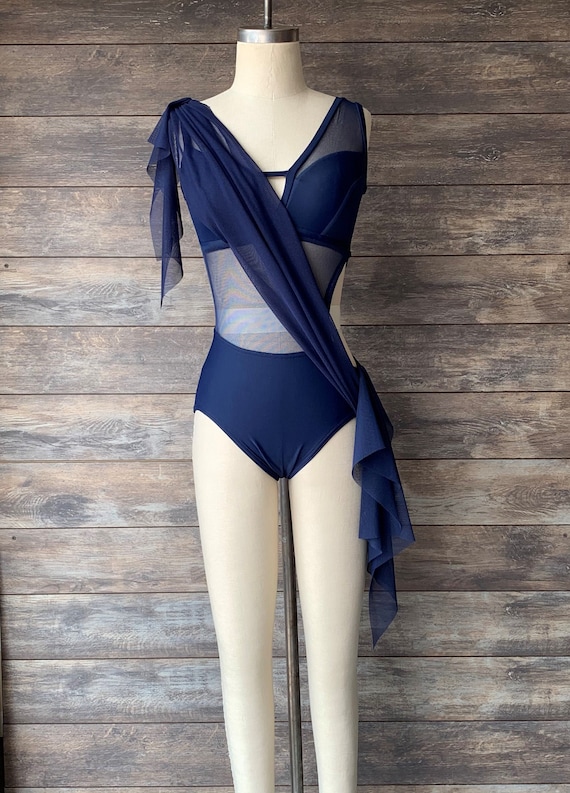This is a detailed photograph of a cream-colored mannequin, displayed in portrait orientation against a light brown wooden shiplap wall. The mannequin, lacking a head and arms, is propped up by a silver metal pole attached at the neck area. It is dressed in a stylish dark navy blue leotard-style bikini featuring a sheer midsection and a deep V-cut neckline. The outfit is accentuated by a floaty sash that ties at the left shoulder, drapes across the torso, and secures at the right hip, creating a dynamic look. The wood grain of the wall behind adds a rustic yet sophisticated backdrop to the overall aesthetic.